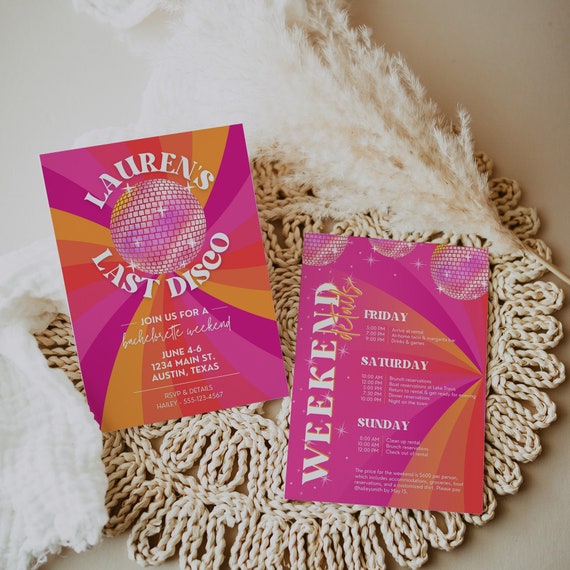This vibrant photograph showcases a meticulously arranged invitation set for "Lauren's Last Disco." Set against a light gray table, the two cards are elegantly displayed on a white knit or lace placemat adorned with feather-like cloth, giving an organic, soft appeal.

The card on the left, representing the front of the invitation, prominently features the title "Lauren's Last Disco" encircling a gleaming disco ball. Beneath it, the text reads, "Join us for a Bachelorette weekend, June 4-6," followed by the address, "1-2-3-4 Main Street, Austin, Texas," and RSVP details indicating, "Hayley, 555-123-4567." The background is richly designed with a dynamic pattern of purple, orange, and yellow sunrays, radiating a 70s groovy vibe.

The card on the right details the event itinerary, marked with the heading "Weekend details." It lays out a schedule for Friday, Saturday, and Sunday, each day featuring distinct activities planned for the bachelorette party. The colorful sunray backdrop continues, while three shining disco balls embellish the top of the card, maintaining the vibrant and festive theme.

This intricate and vividly colored invitation set is stylishly presented on an organically textured placemat, complementing the festive and joyous nature of the event it represents.